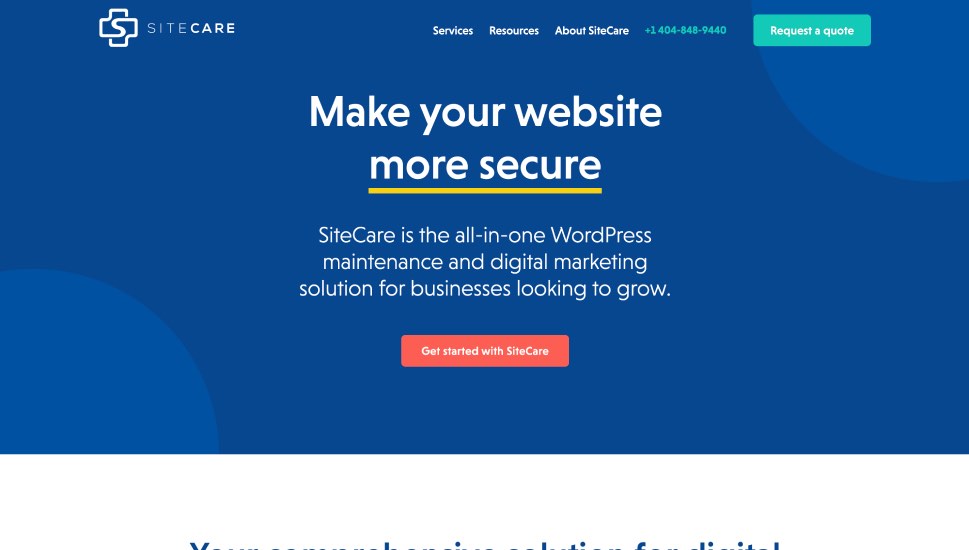**Detailed Caption:**

The image depicts a low-quality, grainy, and pixelated website interface related to a company named "Site Care." The layout features multiple elements organized in a structured manner:

- **Top Line:** The top line displays navigational links in a cross-like pattern labeled "Services," "Resources," "About," and "Site Care."
- **Background:** The overall background of the page is light blue.
- **Primary Rectangle:** In the center, there's a main rectangular section also in light blue, which includes various numbers such as "1, 4, 3, 8, 4, 8, 10, 9, 4, 4, 0."
- **Side Panel:** On the right side of this rectangle, there is text or an indication to "close," presented in small white text, possibly as a button or link.
- **Headline:** The headline "Meet your website. More secure," is underlined in yellow and located prominently on the site.
- **Content Area:** The main body of the content describes Site Care as "the all-in-one WordPress maintenance and digital marketing solution for businesses looking to grow" in white text on the right. 
- **Call to Action:** Beneath this description, a prominent red rectangle with white text urges visitors to "Get started with Site Care."
- **Visual Elements:** The design also includes half-circle shapes, one in the bottom left and one in the bottom right of the background.
- **Miscellaneous:** The bottom area of the image has additional, less coherent text, which may be part of the pixelation issue mentioned.

Overall, the visual elements and text positions seem haphazard due to the image's poor quality and pixelation, making it challenging to discern further details.